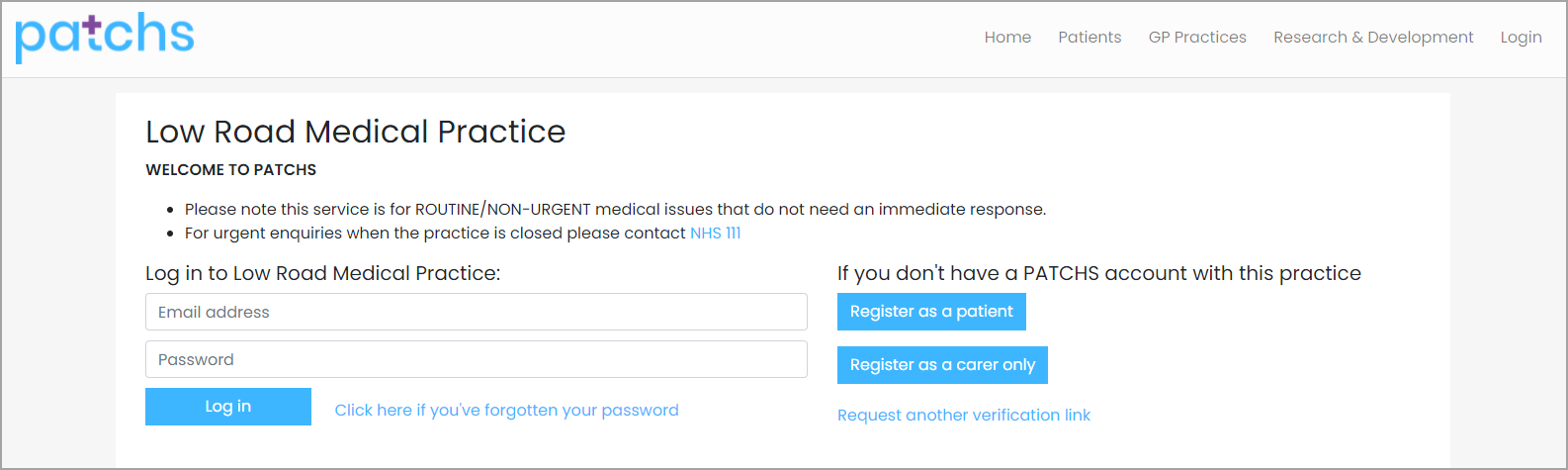This is a detailed screenshot of a webpage with a clean white background. At the very top, there is a white navigation bar. On the left side of this bar, the word "Patches" is displayed in blue font, with the distinctive detail that the cross-part of the letter "T" is rendered in black, resembling a small black addition symbol above the "T." 

On the right side of this navigation bar, there are clickable options presented in gray font: "Home," "Patients," "GP Practices," "Research and Development," and "Login." Each of these can be selected to navigate to the corresponding sections.

Beneath this navigation bar, there is a prominent white rectangle containing the main content. At the top of this rectangle, "Low Road Medical Practice" is written in black font. Below this, a welcome message reads: "Welcome to Patches. Please note this service is for routine/non-urgent medical issues that do not need an immediate response. For urgent inquiries, when the practice is closed, please contact NIIS 111."

Further down, the text "Login to Low Road Medical Practice:" introduces two input fields where users can enter their email address and password. Beneath these input fields, there is a blue button with "Login" written in white font, providing a clear call to action for users to log in to their accounts.